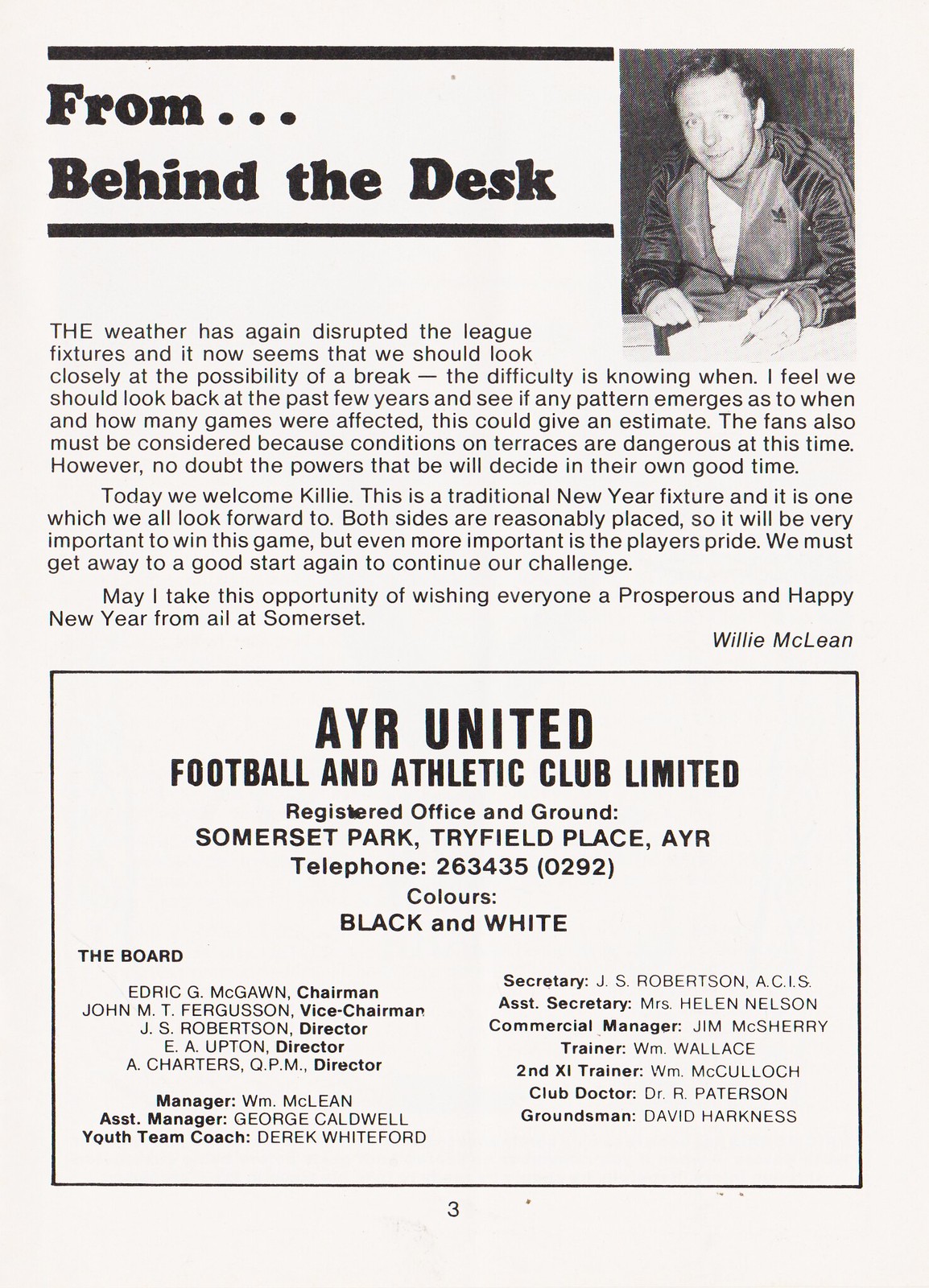The image is a black and white photograph from a newspaper article titled "From Behind the Desk," located on page three of what appears to be an old magazine or booklet. It features a Caucasian man with brown hair, wearing a sports jacket that extends to his wrists. He is holding a pen in his left hand and staring directly at the camera with a slight smile. 

The article discusses the disruption of league fixtures due to weather conditions and emphasizes the need to examine past years for patterns in game cancellations to inform future decisions. It highlights the importance of considering fan safety due to dangerous conditions on the terraces and mentions that the ultimate decision will rest with the powers that be. Additionally, the article notes today's match with Killy as a traditional New Year fixture, stressing the importance of a strong start for the team's continued success and expressing well wishes for a prosperous New Year from everyone at Somerset.

At the bottom of the page, there is a boxed advertisement for Ayr United Football and Athletic Club Limited, listing the registered office and ground at Somerset Park, Trifield Place, Ayr, along with a telephone number. It also mentions the team's colors, black and white, and provides a detailed list of board members, including positions like chairman, vice-chairman, directors, trainers, and the club doctor.